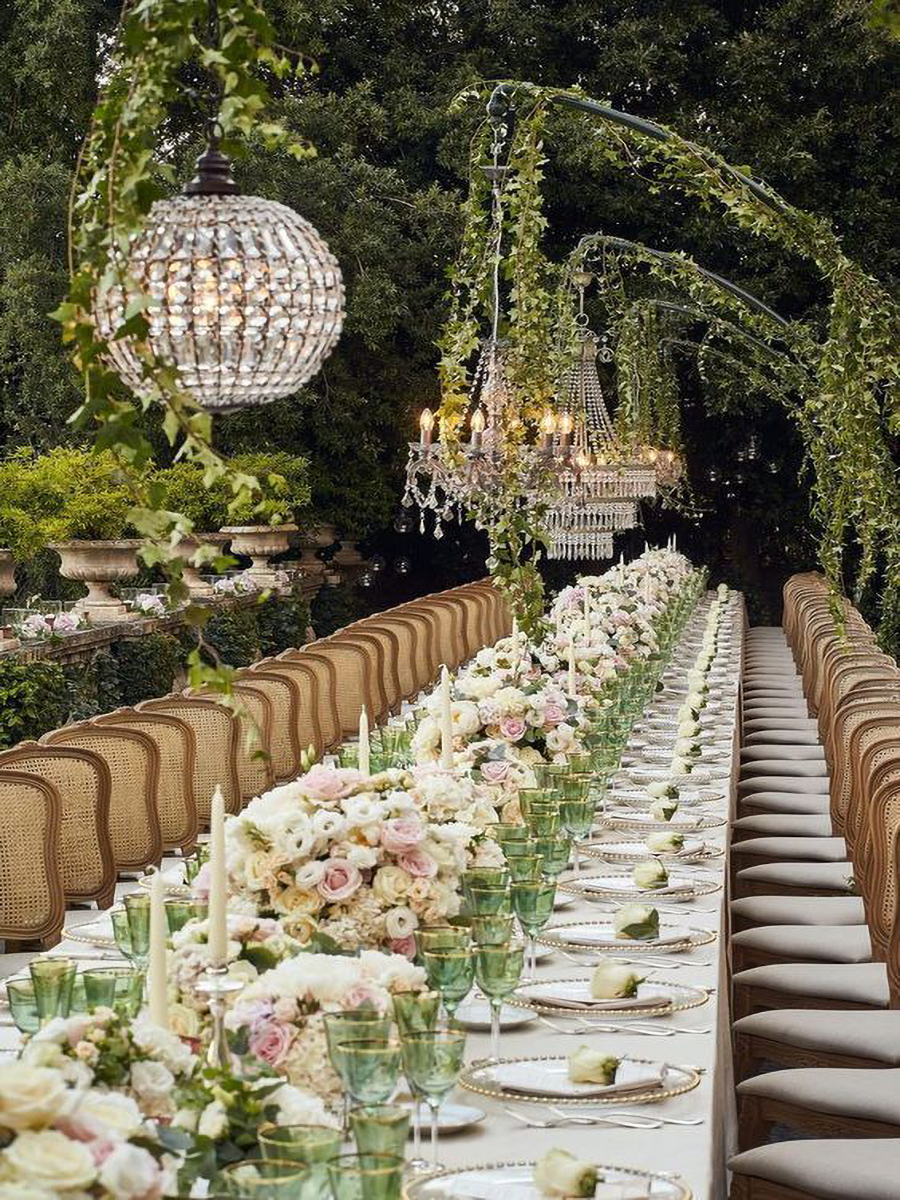This photograph showcases a meticulously arranged outdoor tablescape, likely set for a grand wedding reception or a major celebration in a verdant garden setting. The long, rectangular table, swathed in white linen, extends as far as the eye can see, adorned with a continuous floral centerpiece of abundant pink, white, and beige roses interspersed with white taper candles in elegant silver candlesticks. Alongside the flowers, clusters of green wine goblets glisten, adding a pop of color to the elegant setup.

Each seat at the table is marked by a place setting that includes clear glass chargers with gold beaded edges, stacked with a small white plate delicately holding a white rosebud, exemplifying attention to detail. Silver cutlery is neatly placed beside each setting, with pairs of forks positioned to the left. The chairs are arranged at a slight angle and feature tan wicker backs with beige cushions, enhancing the sophisticated atmosphere.

Above the table, three elaborate chandeliers hang from ivy-wrapped poles, adding a touch of grandeur. There is a variety of chandelier styles, including a large multi-tiered crystal chandelier, a traditional crystal chandelier adorned with leaves, and a round crystal chandelier—all seamlessly blending with the garden's natural beauty. Concrete planters with lush plants are visible to the right, while ivy-covered surfaces frame the bottom left, enhancing the lush, green background that completes this opulent outdoor dining experience.